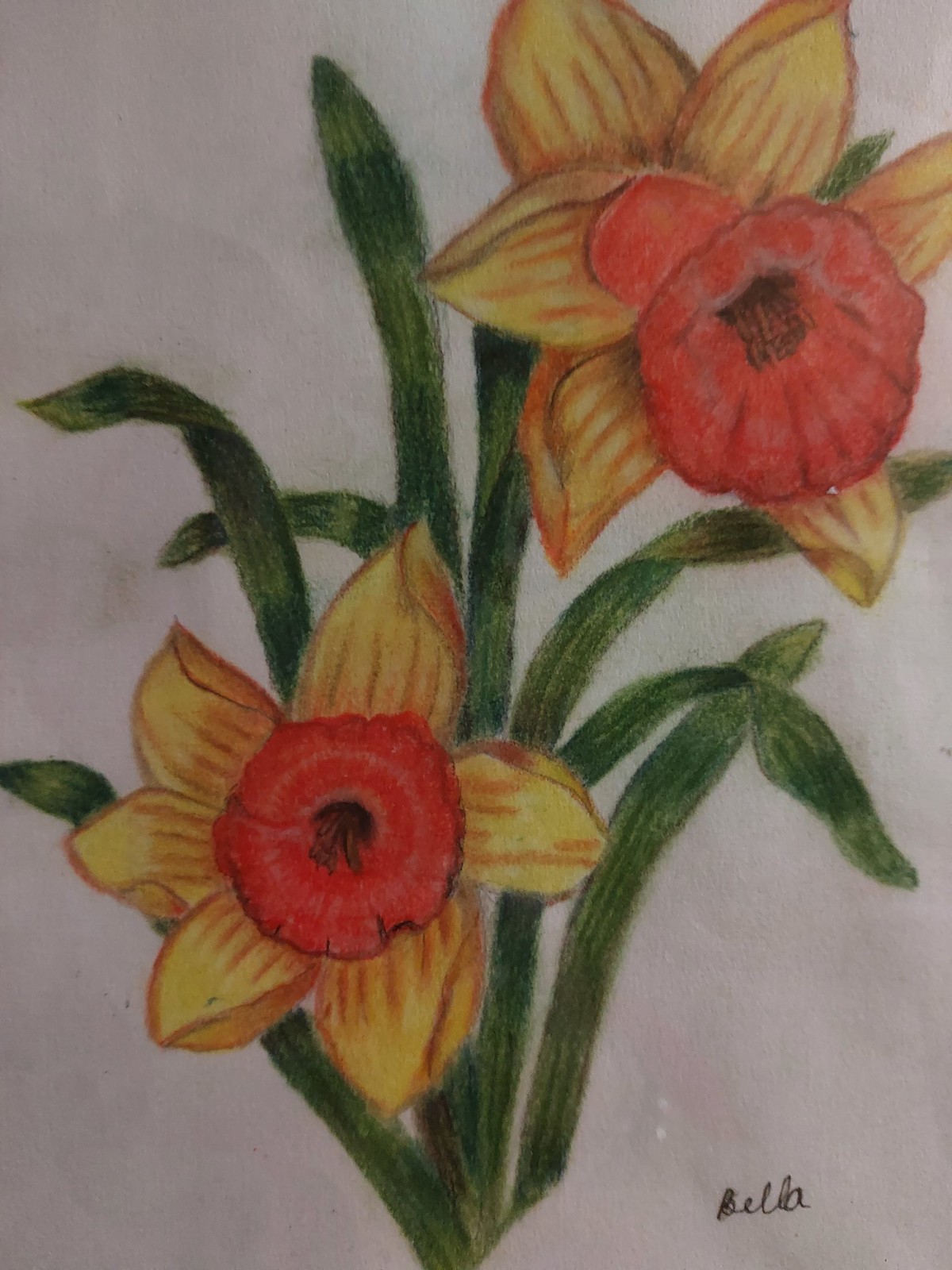This image showcases a portrait-oriented painting featuring two vibrant yellow flowers, each possessing large, pointed petals and an orange circular core at their centers. The painting, signed by the artist Bella in the lower right corner, beautifully captures the juxtaposition of these two blooms. The flower on the right rises higher in the composition, positioned in the upper right corner and gracefully drooping. In contrast, the flower on the left is depicted from a direct frontal view, situated lower in the painting. Surrounding and complementing the flowers are an array of lush green stalks and foliage, which add depth and vitality to the scene. Overall, the detailed nuances and the harmonious arrangement of floral elements showcase the artist's dexterity and attention to detail.